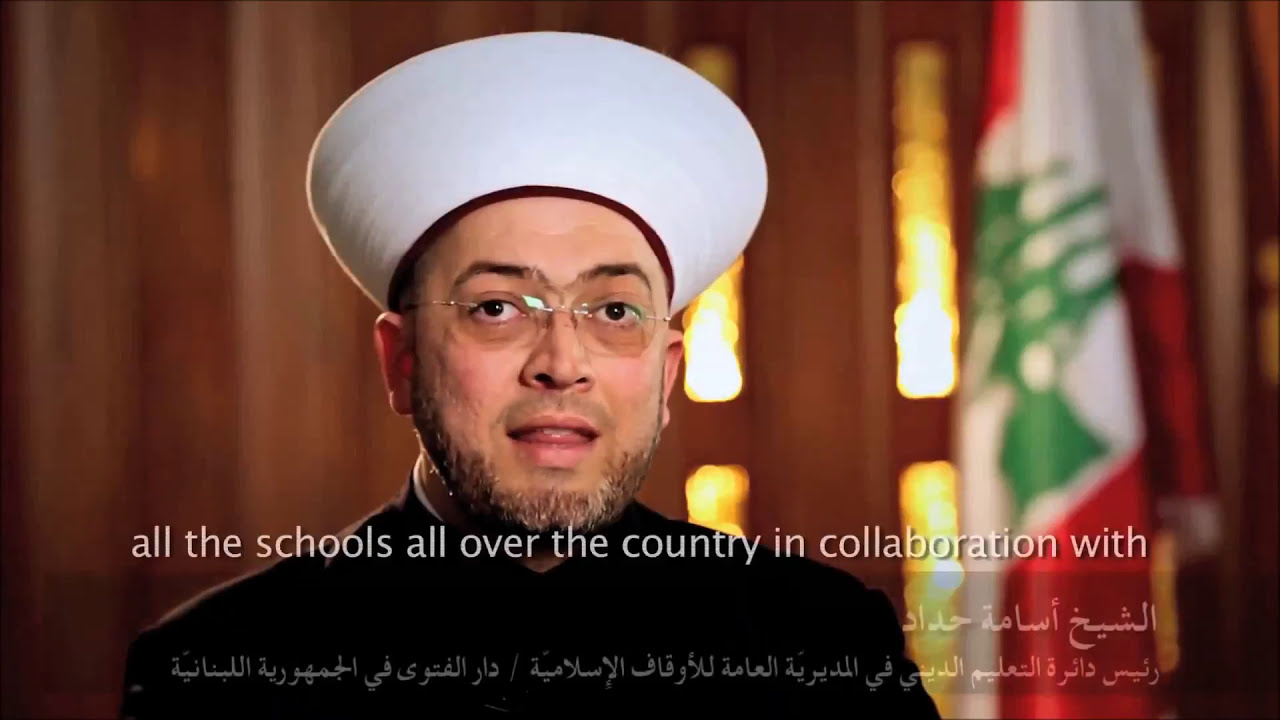In this image, we see a man who appears to be a religious cleric from a Middle Eastern country, possibly Lebanon, as suggested by the red and white flag with a green emblem visible in the background. The man is wearing a distinctive large white hat that resembles an egg in shape, along with a black jacket and glasses. He has a small beard without a mustache and is captured in the middle of speaking, with his mouth open and eyes focused on the camera. The backdrop features what looks like wooden or wood-paneled walls, though it's somewhat blurred, and there are hints of windows letting in light. The scene seems to be either from a news program or an interview, as indicated by the text across the bottom of the screen, which reads, "all the schools all over the country in collaboration with," followed by several lines of Arabic script.